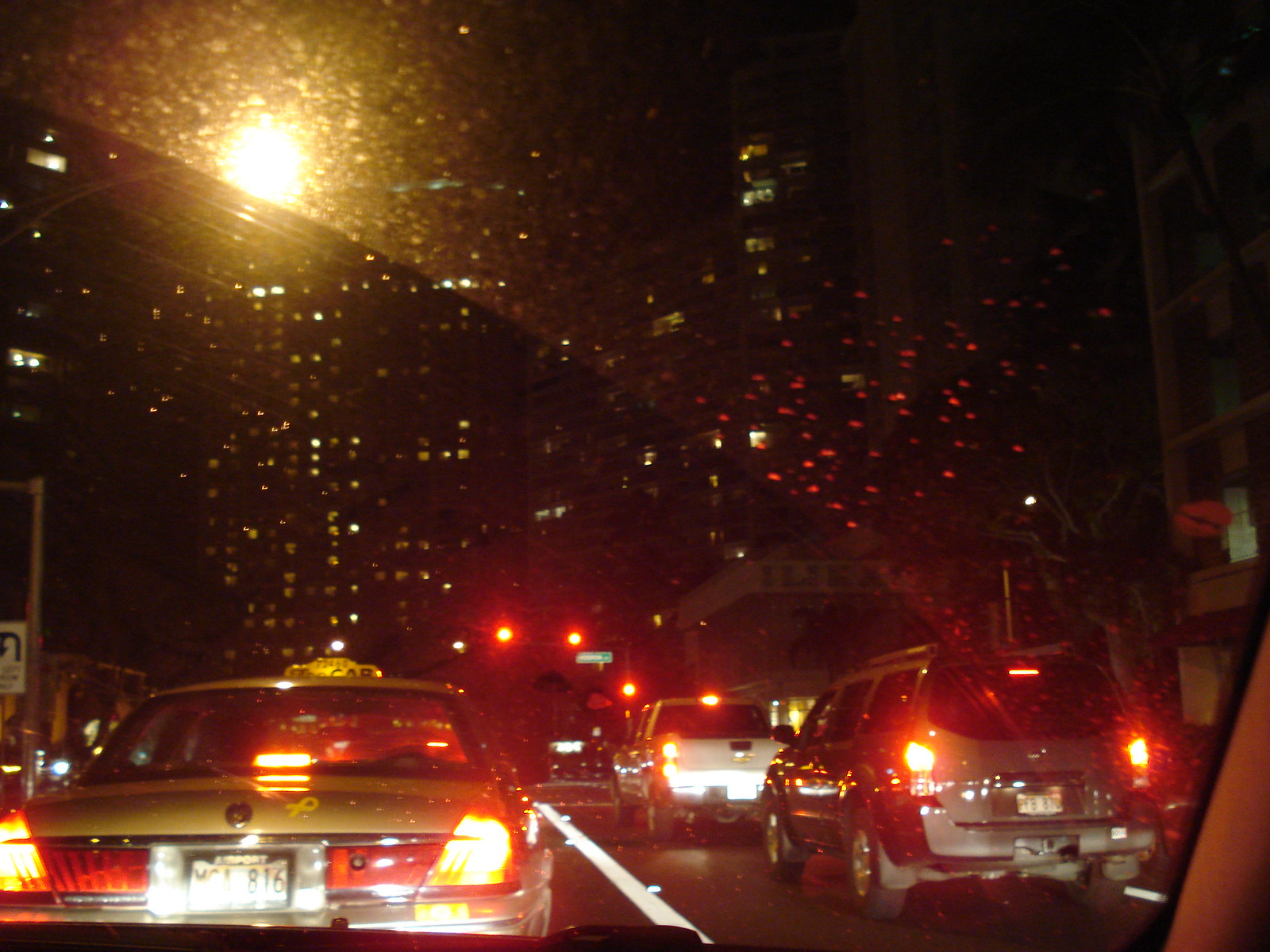This is a nighttime POV shot taken from the passenger seat of a car, looking out the front windshield. The image captures the scene of a densely packed city intersection, where several vehicles, including a yellow taxi directly in front, are waiting at a red stoplight. To the right of the taxi, a white pickup truck and a gray SUV occupy the adjacent lane. The high-rise buildings in the background have their windows illuminated, contributing to the vibrant urban atmosphere.

The windshield of the car, showing a distinctive curved streak from a recent swipe of the wiper, is partly clean but reflects the bright streetlights and the illuminated cityscape, adding a layer of haze to the view. An intense, bright orange light shines from the upper left corner of the photo, possibly from a traffic signal or a lamppost. The sky above is a deep black, dotted with various colored light reflections, giving an impression that it could be drizzling. Above the red traffic light, which dominates the center of the frame, the silhouette of tall buildings and a series of poles can be faintly discerned. Despite the grime on the windshield, the scene vividly portrays the bustling yet paused moment at the city intersection.